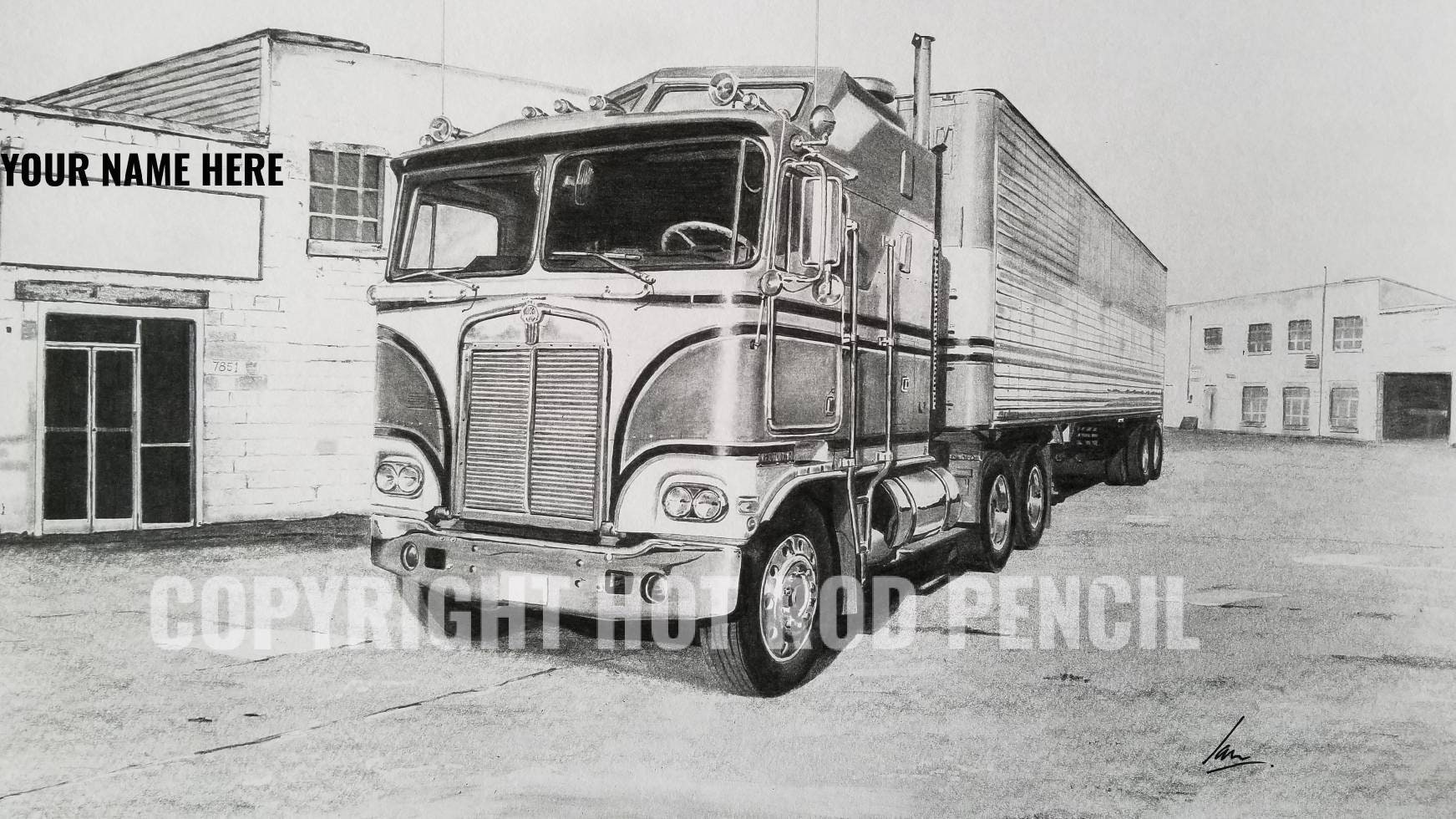The image is a horizontally cropped, grey-toned, monochromatic photograph resembling vintage sepia. It showcases a large semi-truck, possibly an 18-wheeler, prominently placed in the center. The truck's front windshield, grill, and left side of the cab are visible, with its imposing height nearly matching that of the surrounding buildings. In the upper left corner, "your name here" is displayed in black text over a building, which appears to be a block-like factory or business structure with minimal windows. Another smaller building is situated at the middle of the right edge. The clear, well-lit image also features a watermark in the lower third that reads "copyright hot rod pencil," and a signature in black in the bottom right corner. The sky forms the backdrop at the top portion of the image.